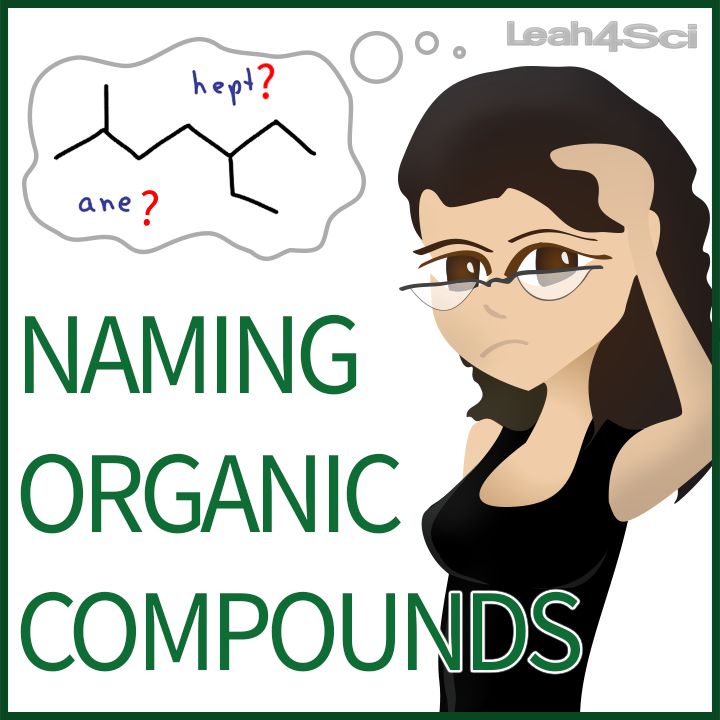This detailed cartoon-like illustration features a young woman named Leah, depicted with light skin, long black hair, and large brown eyes. She is wearing stylish half-rimmed glasses and a black tank top. Leah appears puzzled, holding one hand to her head while pondering a molecular-chemical diagram inside a thought bubble. The diagram includes the annotations "H-E-P-T?" and "A-N-E?" indicating her uncertainty about naming the organic compound. Above her head, the text "Leah 4 Sci" (presumably the creator's identity) is displayed in gray in the top right corner. Additionally, the illustration is bordered in green with large green lettering reading, "Naming Organic Compounds." This meticulously detailed graphic likely serves as a thumbnail or primary image for a lesson-focused content piece on organic chemistry.